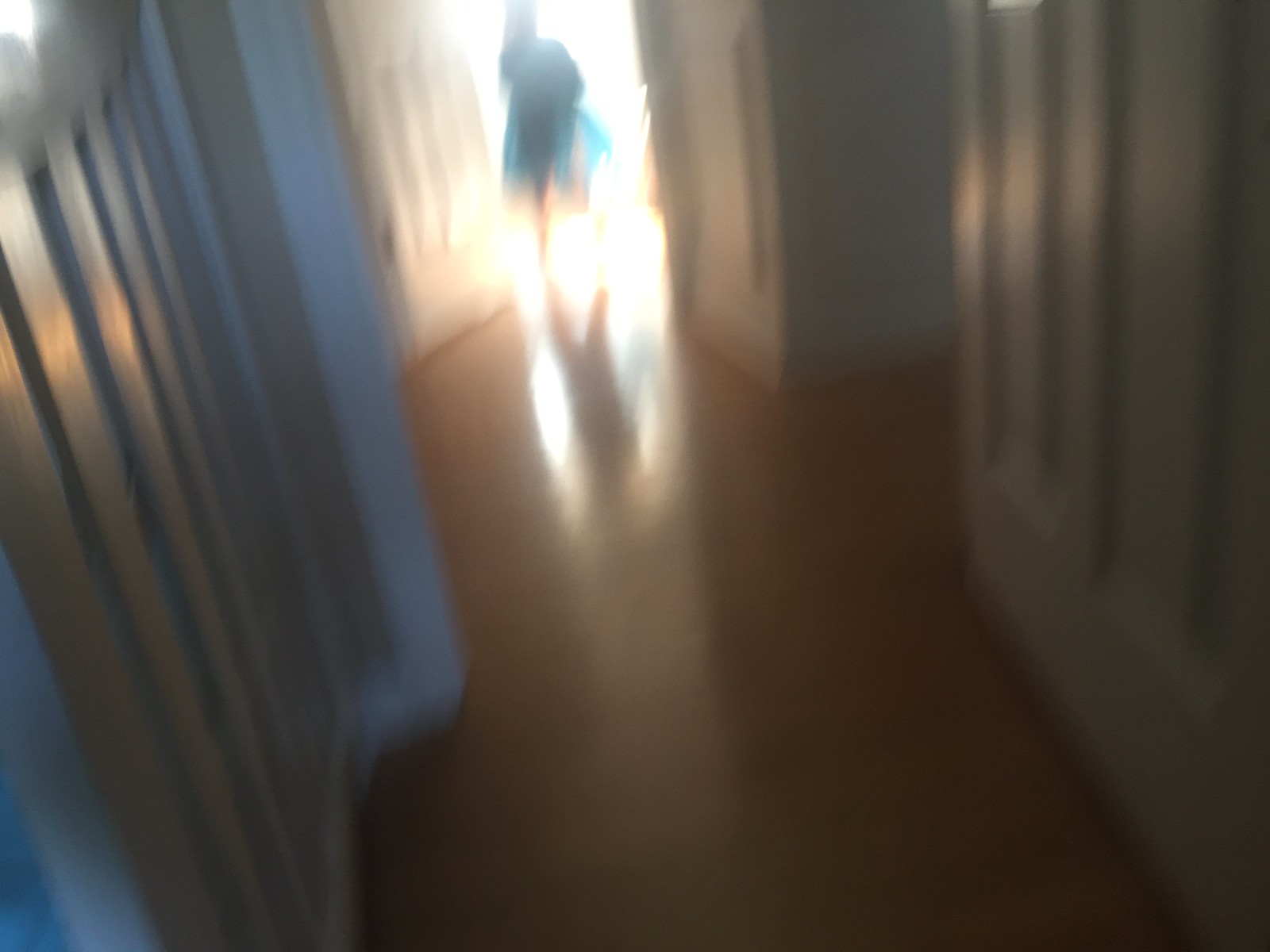A dimly-lit, wooden-floored hallway stretches horizontally within a home, leading the eye to a doorway illuminated by an intensely bright light. The glow is so overwhelming that it nearly obscures the figure standing in the doorway, who appears to be dressed in a blue outfit. The image's low quality and darkened surroundings add a sense of eerie mystery to the scene. On the left side of the hallway, there are a few indistinct white doors and possibly a white pillar, though the details are difficult to discern. To the right, the wall features wainscoting and leads to a turn down another hallway, its path merely suggested by the visible corner. The overall blurred and shadowed ambiance makes it challenging to capture the finer points, enhancing the enigmatic atmosphere of the setting.